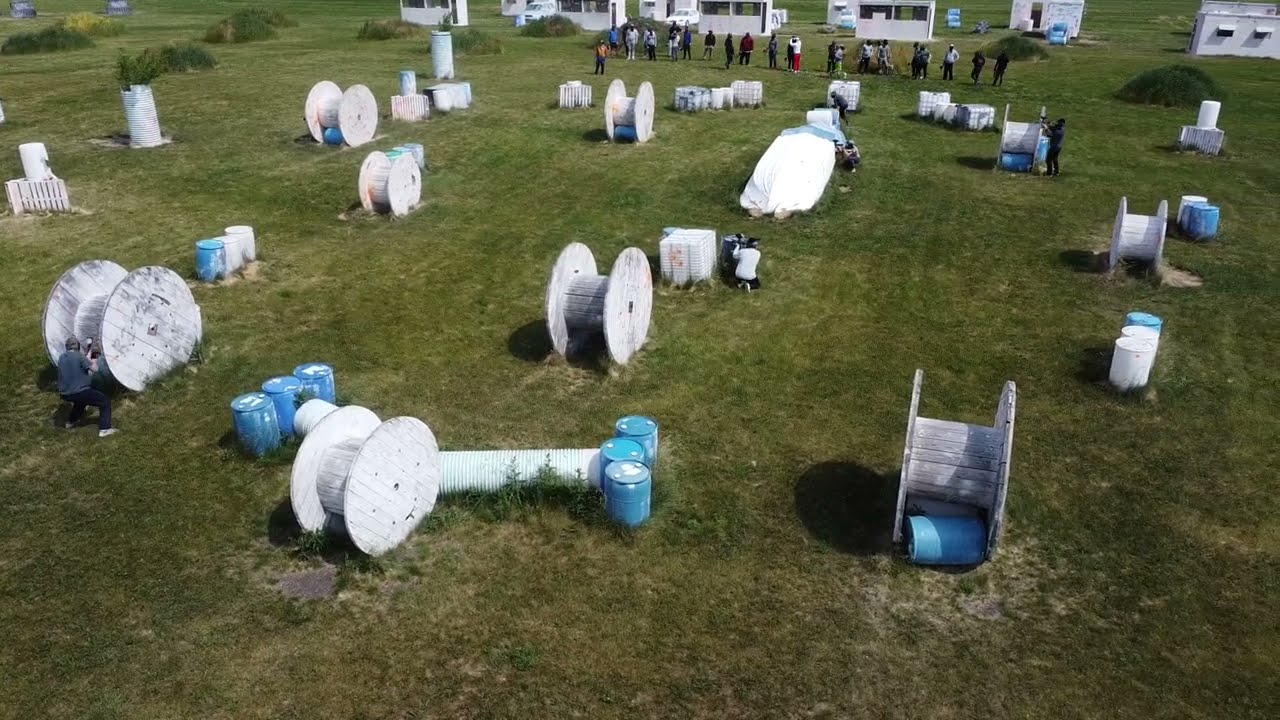The photograph, taken horizontally, depicts an expansive green grassy field scattered with various obstacles, including large wooden cable spools and blue barrels, suggesting the setting of a paintball course or a tactical exercise area. The spools, ranging in size, are positioned throughout the field, with some people crouching behind them. These individuals are dressed in long pants and long-sleeved shirts, and their faces are not visible, adding a sense of anonymity to the scene. 

In the upper center of the image, a group of approximately 10 to 12 people are standing in a line in front of a series of low white structures, which appear to be small outbuildings or kiosks. The scene is set outdoors during daylight hours, with lush green grass and hints of small bushes and darker patches of grass enhancing the vibrant, natural setting. No vehicles are visible, emphasizing the open, uninterrupted expanse of the area.